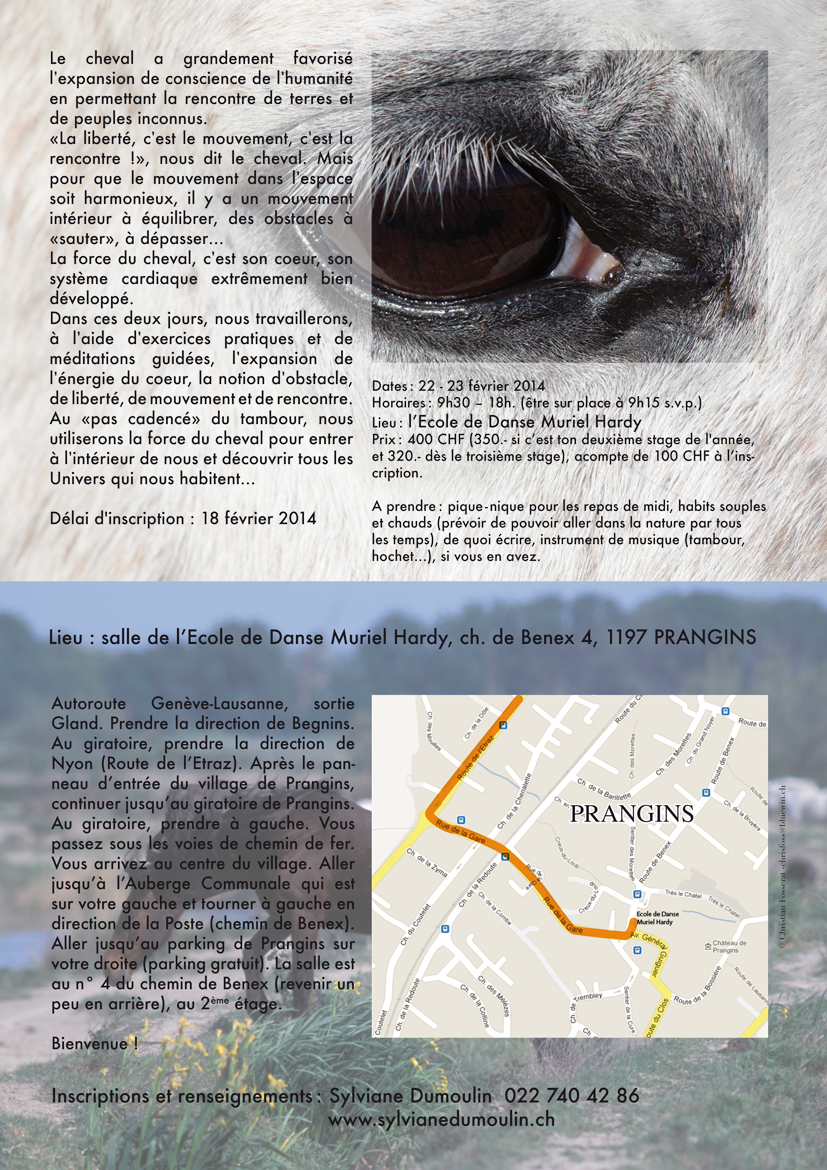The image appears to be from a magazine or encyclopedia page, possibly in French, with substantial amount of small black text both at the top and bottom. The top portion features a highly detailed close-up photograph of an animal's eye, likely a horse's. The horse has white short fur and white eyelashes, with brown eyes and black skin surrounding the eye. This section lies against a greyish background.

The bottom portion of the image shows a blurred outdoor background with a brown horse and highlights a map with orange and yellow lines indicating a specific location. Text near the bottom suggests dates, times, an address, and a website related to Sylvain Dumas. The outdoor scene is likely a field or forested area. The primary heading of the map mentions "Prangins," and the text includes phrases suggesting event details or a schedule, possibly for February 2014. The information implies this is part of a detailed article or advertisement targeting a French-speaking audience.